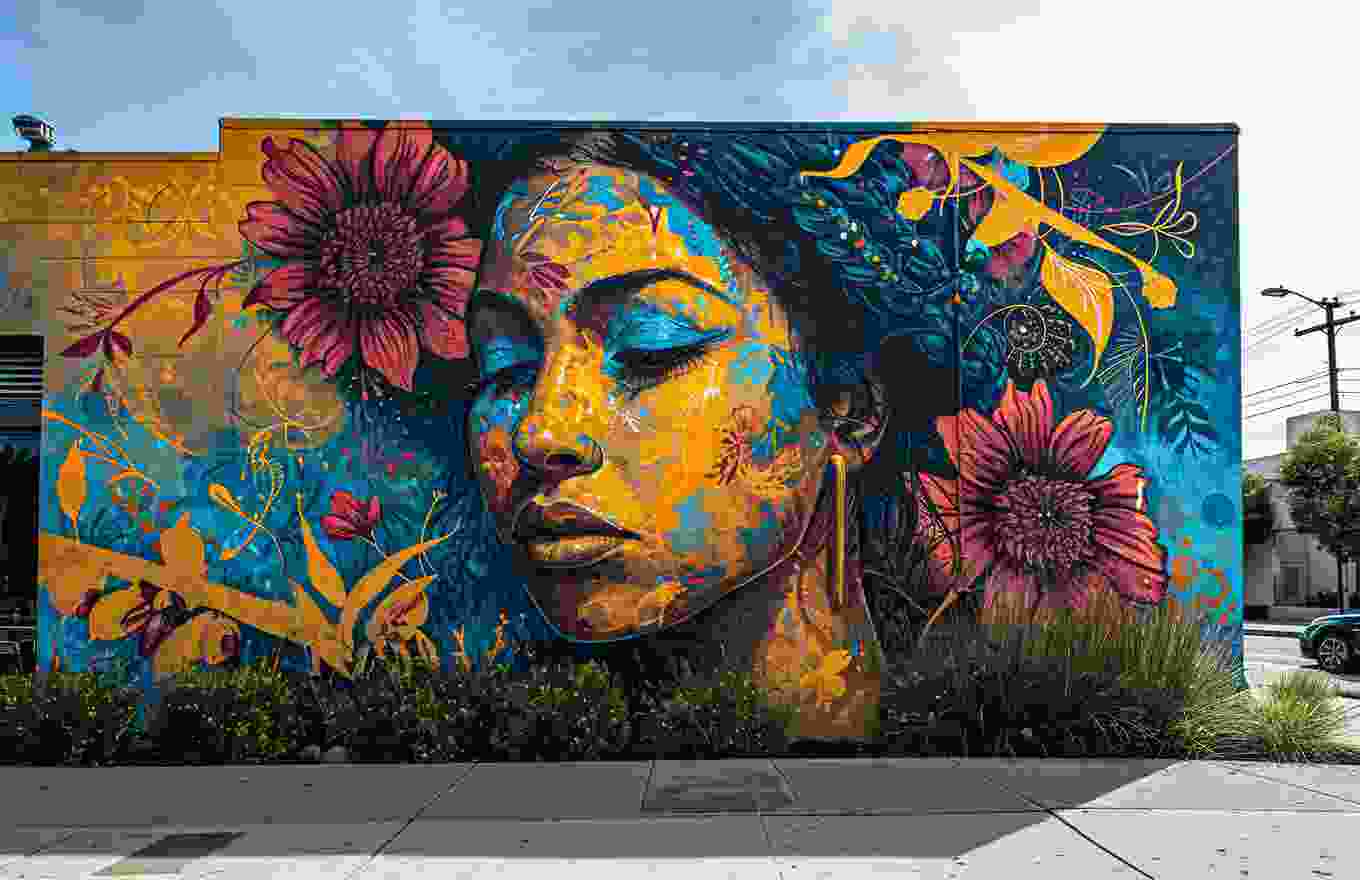The image showcases a highly detailed and artistic piece of graffiti on the side wall of a building in a barrio neighborhood. The mural features a stunning young woman with blue eyelids and her eyes gently closed, revealing long eyelashes. She has full lips, a narrow nose, and sports a dangly earring. Her hair is black, adorned with beads, adding to her elegant appearance. She has a unique yellowish skin tone and is depicted with blue, turquoise eyeshadow.

Surrounding her head are graffiti flowers with darkish red petals, and additional graffiti elements depict yellow plant leaves in the top corners of the mural. The wall itself is composed of cinder blocks, adding an urban texture to the artwork. Alongside the wall, there are shrubs, mulch, and a partially visible car adjacent to a gray sidewalk. The setting includes a street with a light pole and trees, under a sky that appears pixelated with shades of blue and scattered clouds. Overall, the image is both vibrant and natural, capturing a blend of artistic expression and everyday street scenery.